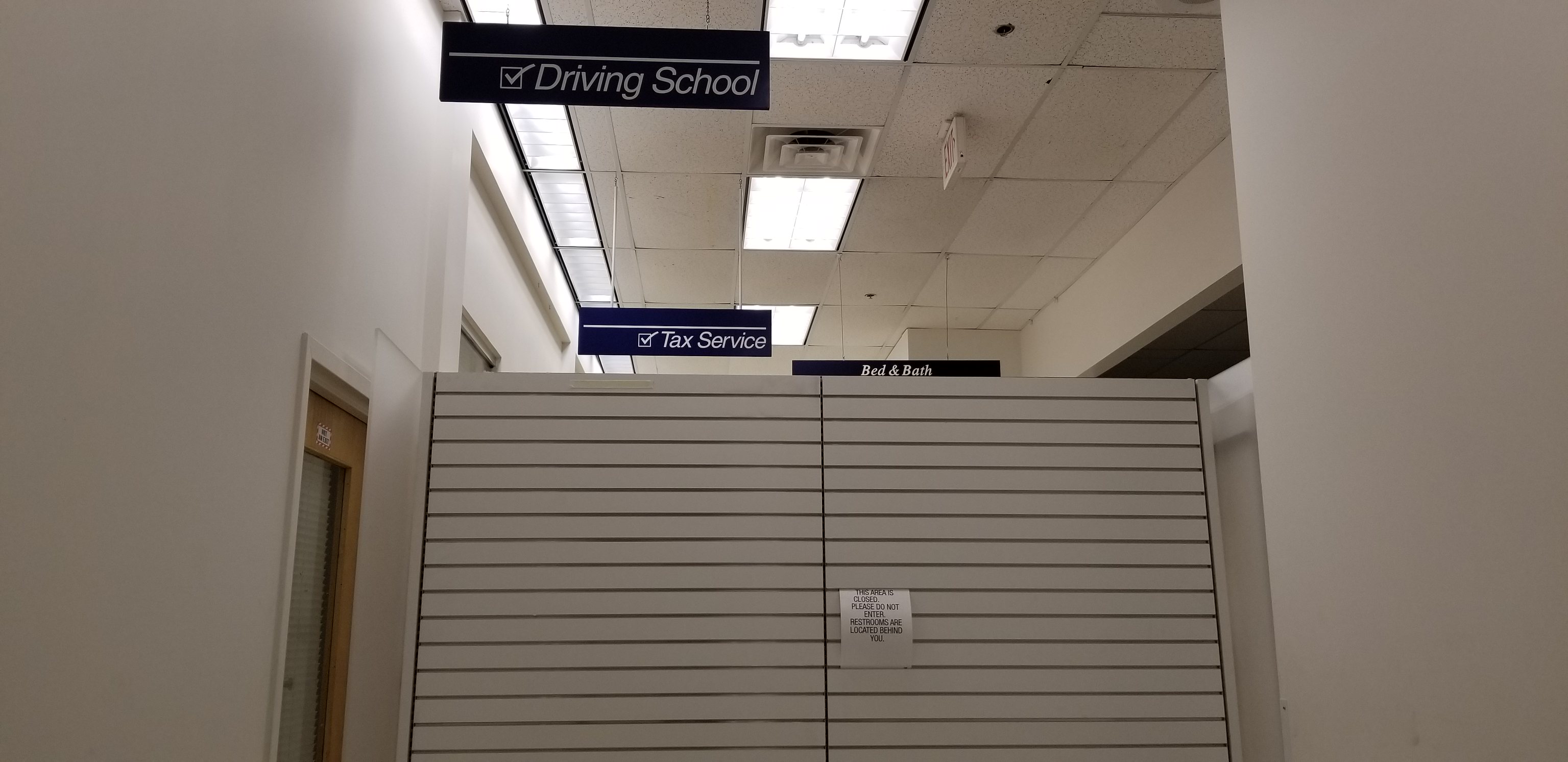This image depicts the interior of a multi-service government facility or office building. Prominently featured are various labeled sections above doorways, indicating different services provided within the building. The entrance labeled "Driving School" boasts a checked-off marker above it, highlighting its operational status. Nearby, a similar checked-off sign reads "Tax Service," suggesting another available service. Further along, a partially visible sign labeled "Bed and Bath" is seen, though the lower part of this section remains obscured. The environment is characterized by white walls and a door with a brown trim and a central glass pane, contributing to the functional yet straightforward aesthetic. Additionally, a wall equipped with horizontal lines, possibly for holding receipts or documents, emphasizes the organized nature of this facility.